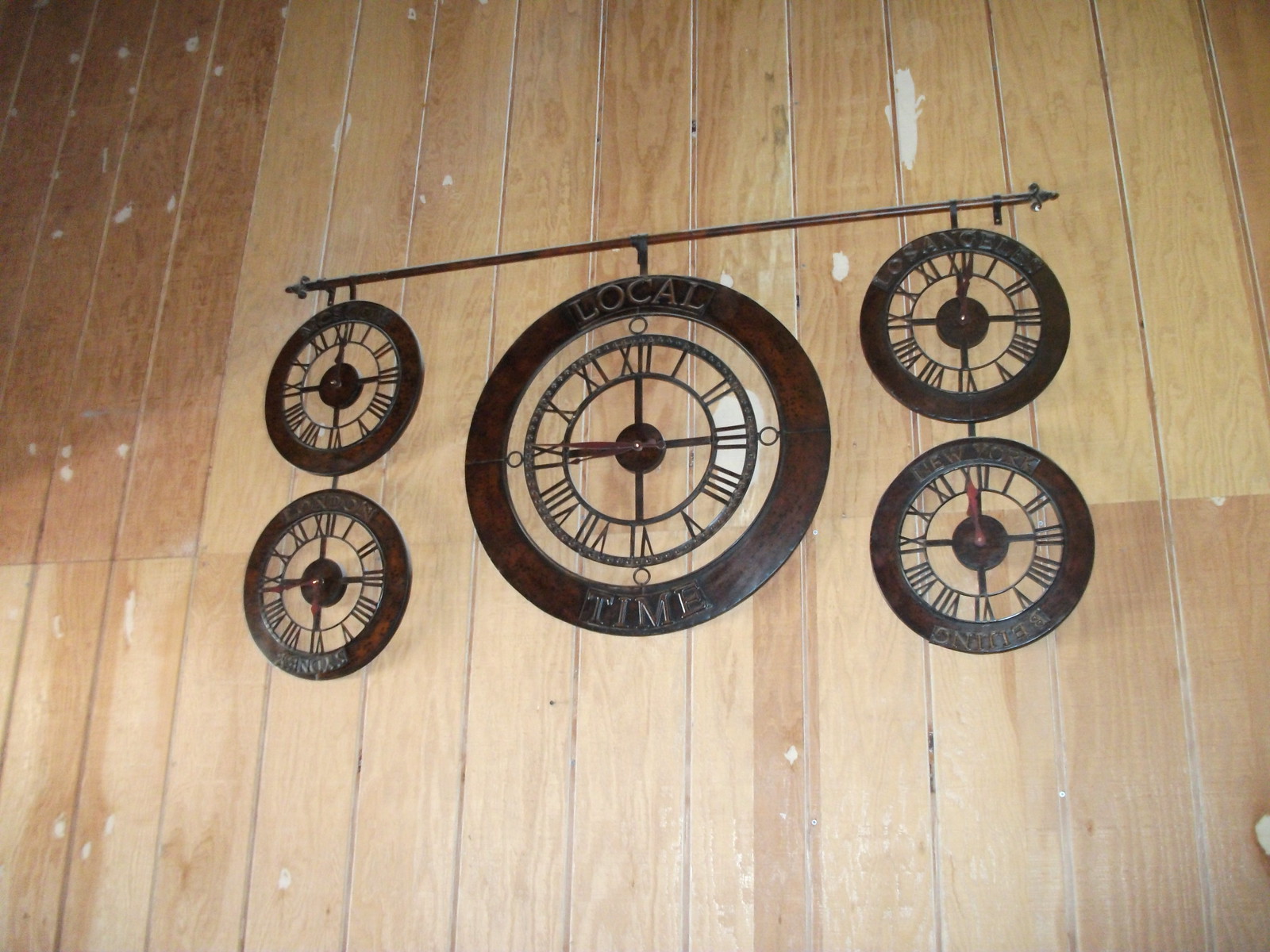This image features a visually captivating arrangement of five dark metal clocks mounted on a vertically paneled, distressed wooden wall. At the center is a prominent, large round clock made to look aged with dark brown and black hues. The clock's face showcases Roman numerals connected by a series of small rings, with a wide outer ring linked by four smaller circles. Raised letters at the top and bottom of this clock read "Local" and "Time." The clock's hands indicate it is around a quarter to nine. Flanking the central clock, two pairs of smaller clocks hang from what appears to be a copper bar or curtain rod. These smaller clocks share a similar Roman numeral design but lack the connecting circles found on the central clock. The clocks on the right are labeled "Los Angeles" at the top and "New York" below, while on the left, one says "London" at the bottom, and the top clock has an indistinct label, possibly "Moscow." Each clock displays a different time, suggesting they represent various time zones, but it remains ambiguous whether they are functional or merely decorative. The distressed wood paneling with its vertical grain adds to the overall rustic and weathered aesthetic of the scene.